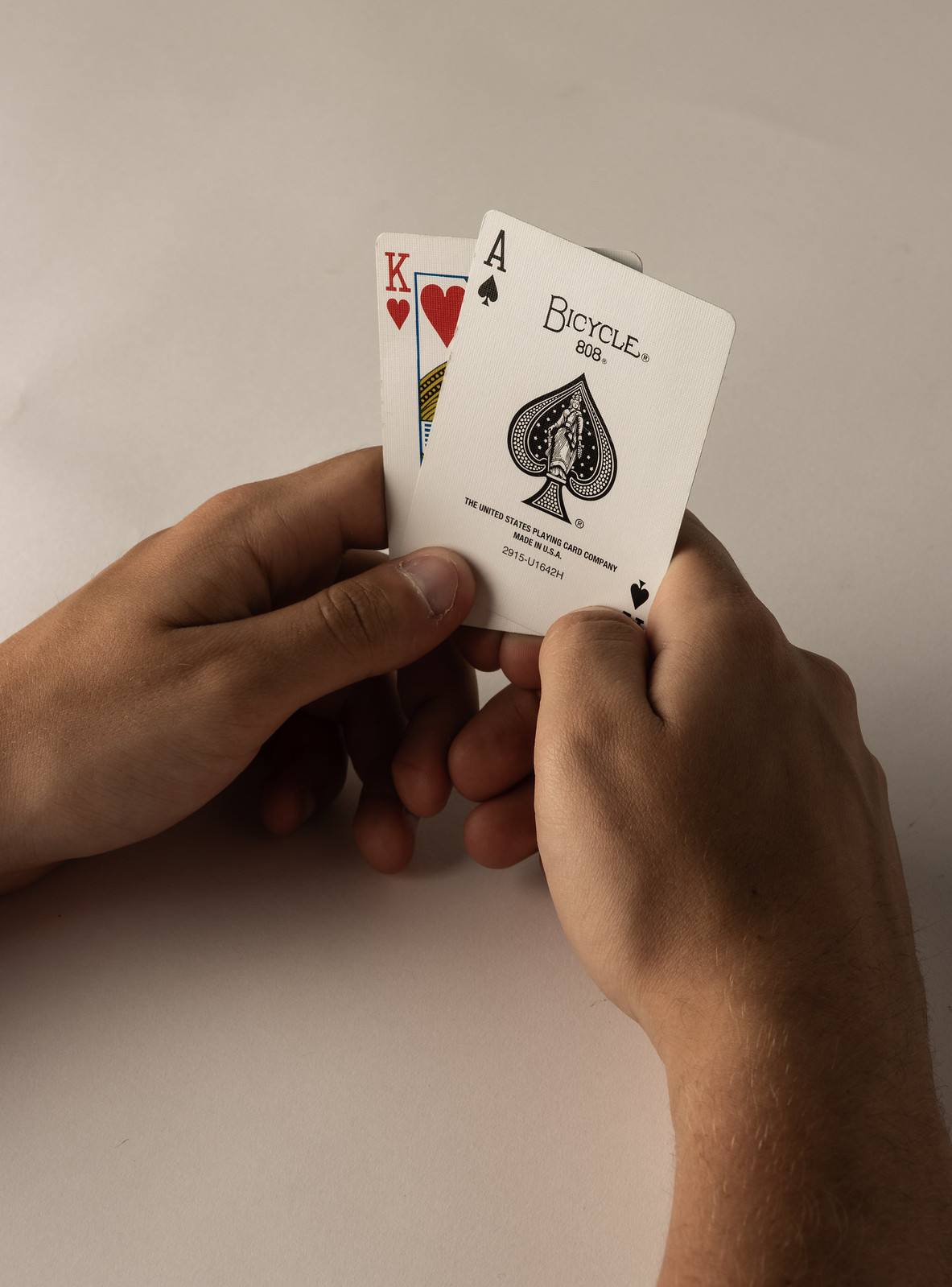The image features a vertical rectangular background with a subtle blend of varying shades of gray. The interplay of shadows and light creates an illusion of depth, giving it a slightly textured appearance, as though different grays are merging together. Upon closer inspection, there are a few subtle wrinkles or creases, resembling the effect of someone pressing their hand against a smooth surface, possibly paper. These creases are more noticeable in two specific areas, though the texture appears to smooth out towards the bottom.

In the foreground, two hands are visible. The left hand is fully seen, while only the wrist and a portion of the forearm of the right hand are visible. Each hand grasps a playing card. The card in the left hand is the King of Hearts, while the card in the right hand is the Ace of Spades. Both cards appear to be from a Bicycle deck.